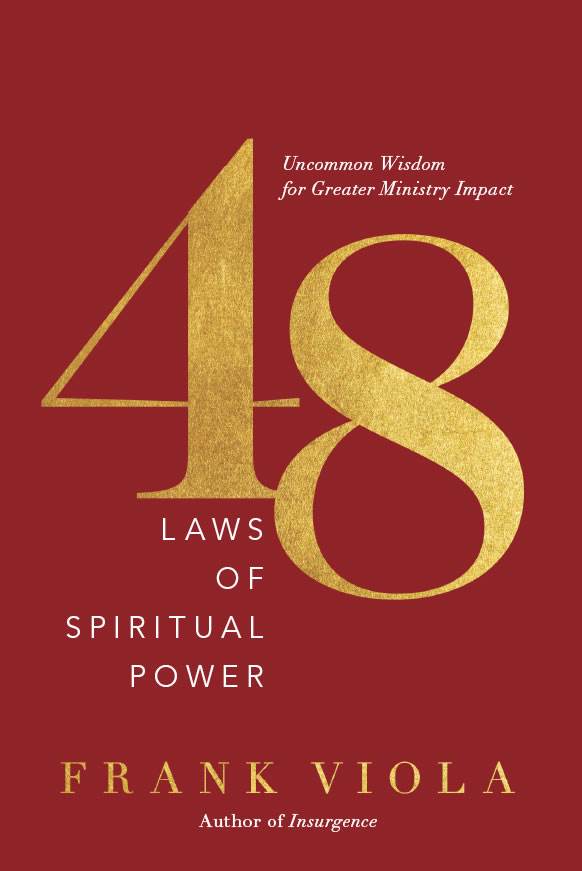The cover of the book features a dark maroon background with a large, striking gold "48" centrally positioned, where the "4" is slightly elevated and the "8" descends to the right. Situated in the upper right corner, the subtitle reads, "Uncommon Wisdom for Greater Ministry Impact," in white lettering, while directly below the number in the center, it states, "Laws of Spiritual Power," also in white. The author's name, Frank Viola, is displayed prominently at the bottom in gold text, and beneath that, in white text, it mentions, "Author of Insurgence."